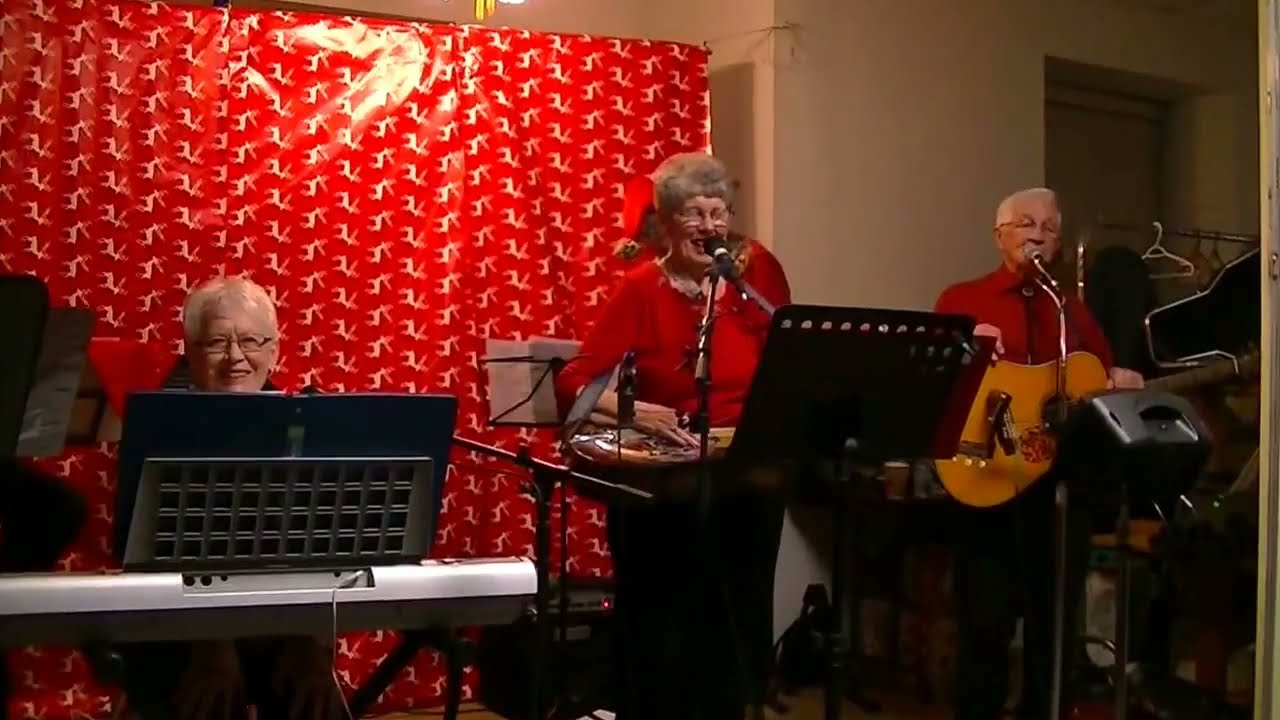The image features a band of three elderly Caucasian individuals performing indoors. The setting includes a woman on the left with white hair and glasses, seated behind a keyboard with an open sheet of music in front of her. In the center, another woman stands, also with gray-white hair and glasses, wearing a red shirt, and is positioned behind a microphone. She appears to be playing an instrument with an open book on a stand before her. On the right, an elderly man with white hair and glasses stands holding an acoustic guitar and singing into a microphone. All three are dressed in red tops paired with black pants. The backdrop behind them is dominated by a red curtain adorned with white designs resembling reindeer, suggesting a Christmas concert theme. There's a visible door to the right along with a clothing rack with hangers and a set of speakers. The walls appear to be white, though slightly dirty, with spiderwebs noticeable in the top corner. A light source positioned between the two women casts a reflective glow on the red backdrop.